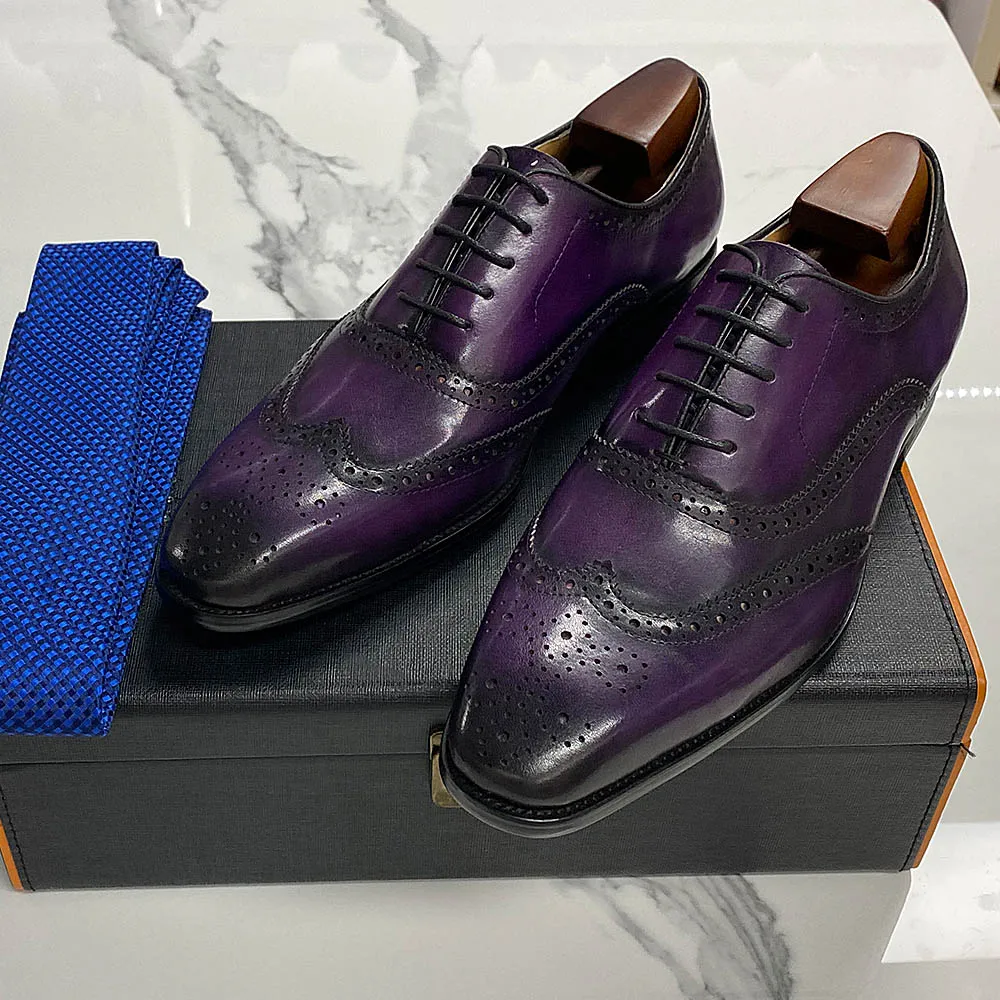In a well-lit room, a pair of meticulously polished, eggplant-colored leather dress shoes are displayed atop a sleek black rectangular box with a metal lock. The shoes, a unique blend of purple that transitions to black at the toes, feature black shoestrings and decorative stitching resembling a W and a wide U just below the laces. Inside each shoe is a wooden support structure to maintain their shape. Adjacent to the shoes on the left side lies a blue tie. The entire setup rests on an elegant, smooth, white marble countertop with grey veining, which reflects the ambient light, giving the scene a sophisticated aura.